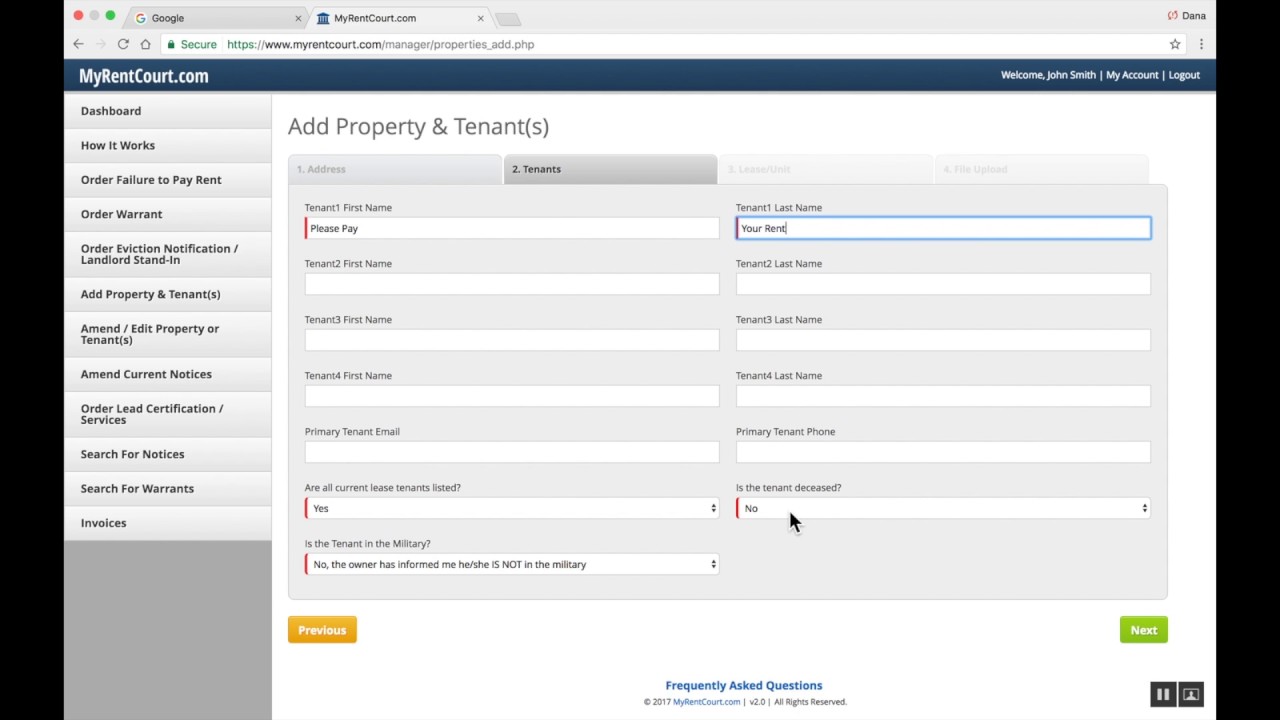A screenshot from MyRentCourt.com, displaying an online form for adding property and tenant information. The user has filled in the form with a humorous, albeit direct message: in the "First Name" field, it says "Please pay," and in the "Last Name" field, it says "your rent." The understated, yet firm reminder exemplifies the creative ways landlords sometimes prompt tenants to fulfill their rent obligations.